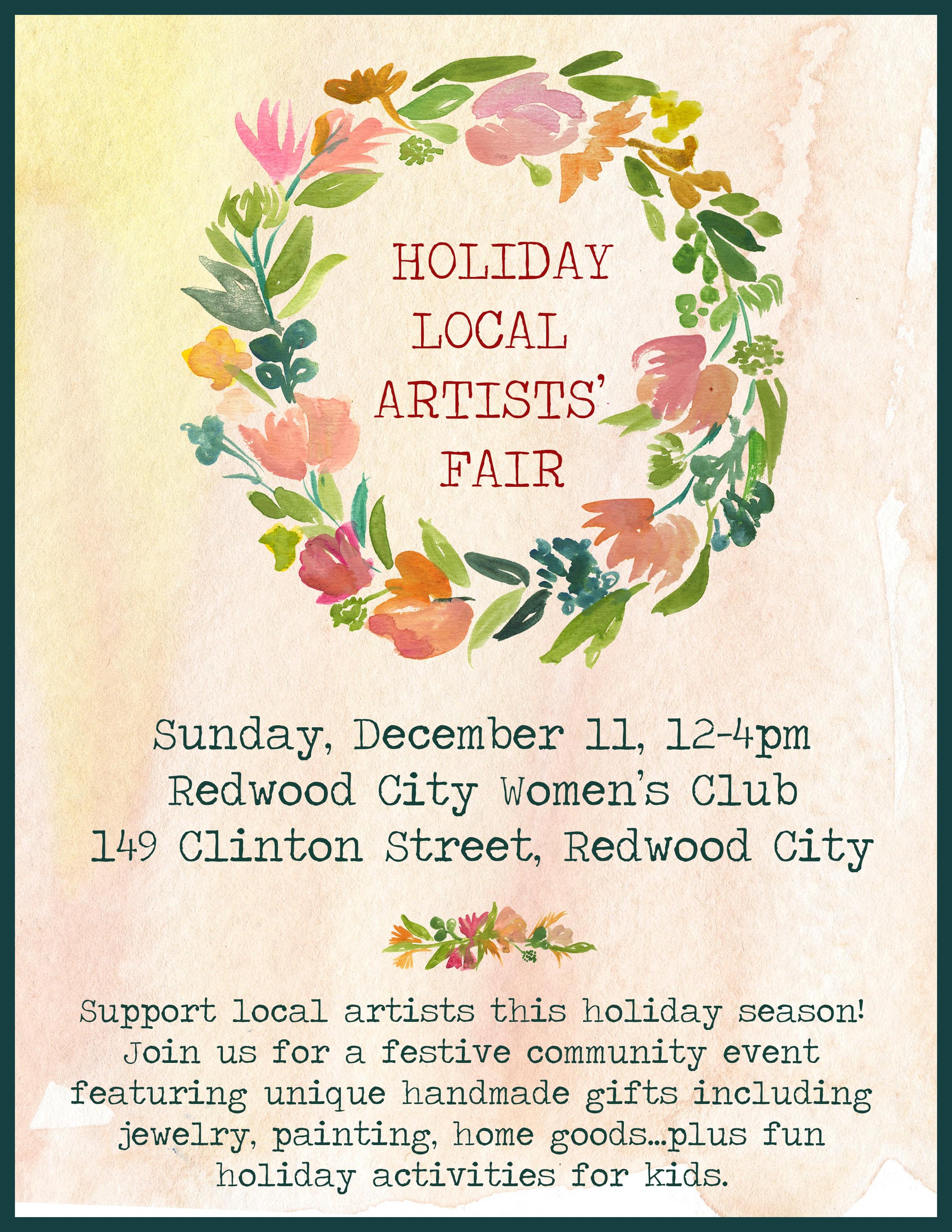The image in question is a painted poster advertising the "Holiday Local Artist Fair." It features a dark black border framing an interior with a light cream, marble-like pattern and a bluish-green trim around the edges. The backdrop consists of a gentle watercolor wash with splotches of light yellow and pink. 

At the top center, the title "Holiday Local Artist Fair" is prominently displayed in dark pink letters, encircled by a vibrant wreath of painted flowers and green leaves, showcasing hues of pink, orange, yellow, and lava pink. Below this wreath, the details of the event are provided in blue lettering: 

"Sunday, December 11th, 12 to 4 p.m., Woodward City Women's Club, 149 Clinton Street, Woodward City." 

Further down, separated by a decorative border of flowers and their green leaves and stems, the poster invites the community with the message, also in blue: 

"Support local artists this holiday season. Join us for a festive community event featuring unique handmade gifts including jewelry, painting, home goods, plus fun holiday activities for kids."

The overall aesthetic of the poster is softened by its watercolor background, creating a warm and inviting feel that reflects the spirit of the holiday season and the community-focused event.